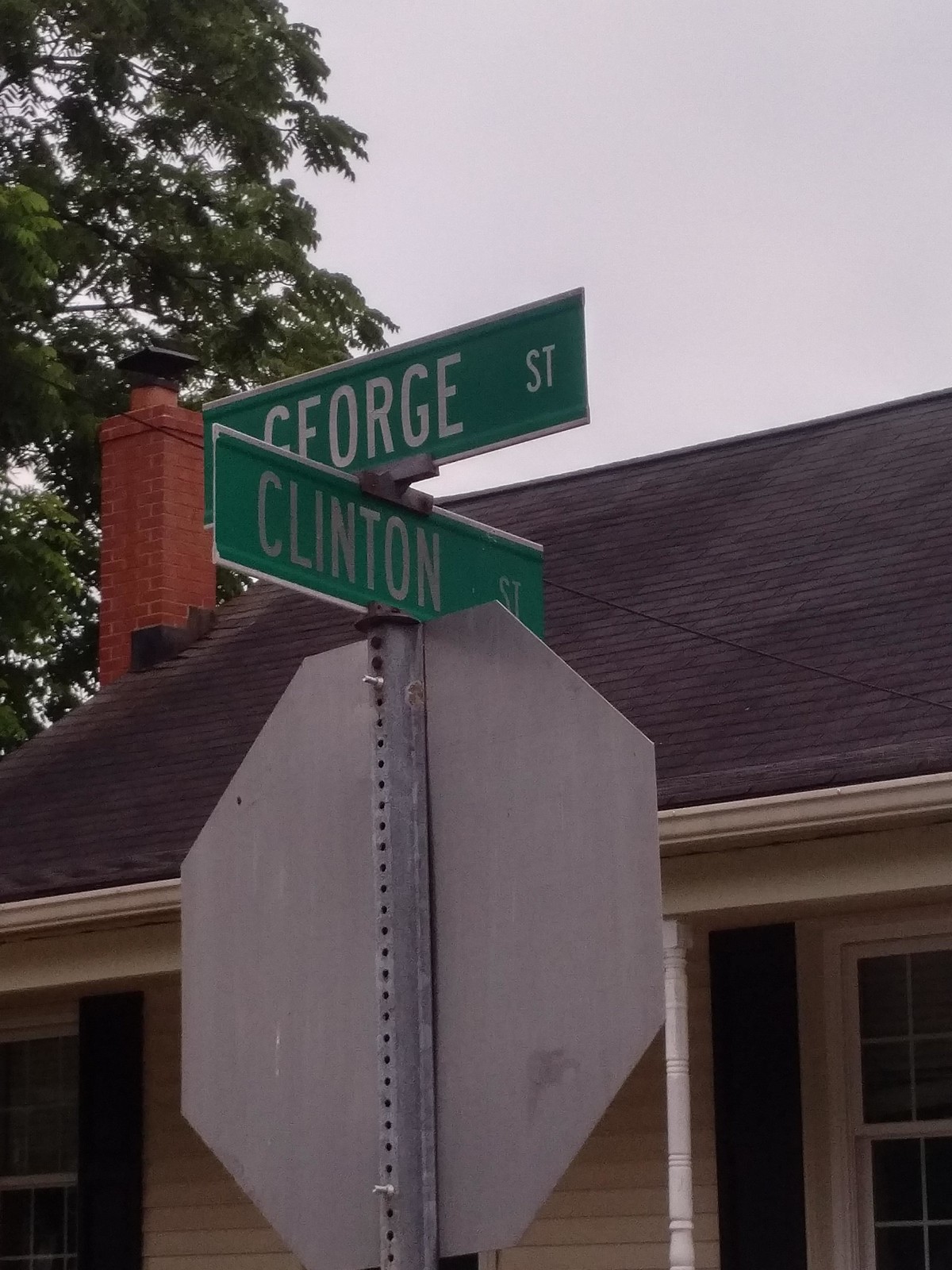The photograph captures a street scene bathed in natural light, dominated by a large, mature tree with lush green leaves in the background. A quaint house with a red brick chimney and a peaked roof peeks from behind the foliage, contributing to a serene residential ambiance. In the foreground, a silver metal pole rises from the ground, supporting an octagon-shaped stop sign, visible only from its reflective silver back. At the apex of the pole, green rectangular street signs intersect, clearly marking the crossroads of George Street and Clinton Street.